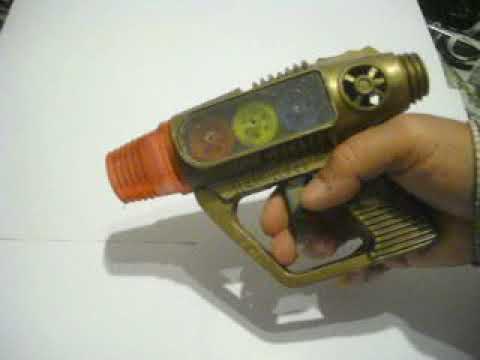The close-up image features a pudgy hand with light brown skin holding a futuristic toy gun, extending from the middle right into the frame. The toy gun, predominantly plastic, boasts an olive or bronze-like color, designed to emulate a sci-fi aesthetic. The tip of the gun showcases a distinctive orange spire. On the side of the toy, a clear plastic compartment reveals three colorful gears—orange, yellow, and blue—arranged side-by-side, suggesting they might spin when the trigger is pulled. The background is a white surface, likely a table, and the scene includes the noticeable shadow of the gun and hand, adding depth to the grainy photograph.